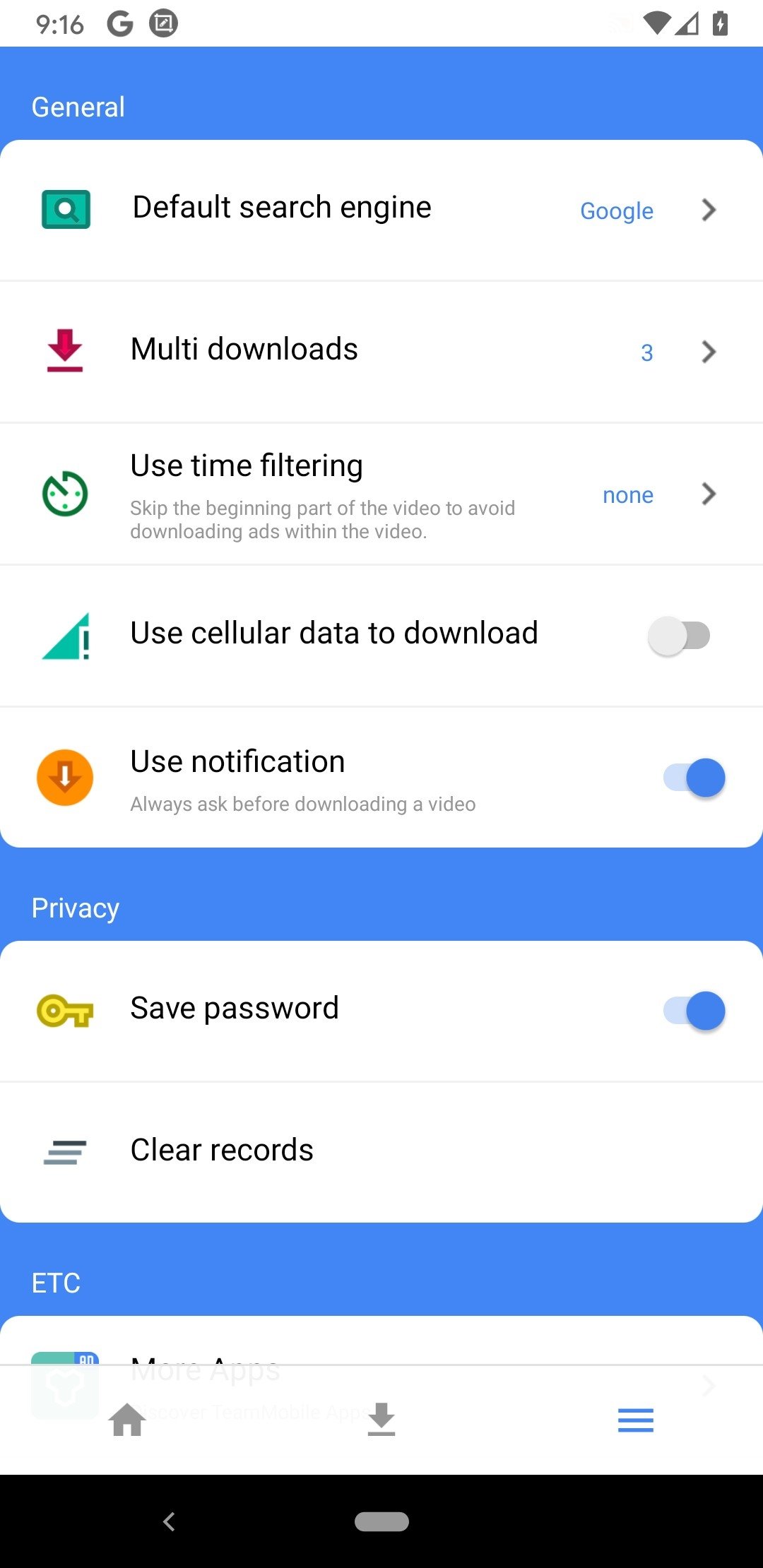This image showcases a smartphone screen capturing various settings and status indicators. At the top right corner, the screen displays a battery icon showing the current charge level, the signal strength bars, and the time, which is 9:16. Additionally, there is a 'G' symbol in gray, likely indicating the mobile network type.

The screen has a blue header with the title "General." Beneath this, there is an option labeled "Default Search Engine," which is set to Google, indicated by an adjacent arrow. Below this setting is a section on "Multi Downloads" featuring a red arrow pointing to a text reading '3 in blue,' along with a red line. Additional settings within this section include "Use Time Filtering," denoted by a clock icon and showing "none" with an arrow beside it; "Use Cellular Data to Download," marked by a green triangle but currently grayed out; and "Use Notification," represented by an orange circle with a down arrow and enabled in blue.

Further down, there is another blue section titled "Privacy." Within this section, the "Save Password" option is highlighted with a golden key icon and is turned on. There is also an option labeled "Clear Records," featuring three lines next to it, and an additional label "ETC" in blue, which appears partially cut off, suggesting more settings are available upon scrolling.

The image also includes the top edge of a green box below this section, and the black line at the bottom edge of the phone, indicating the end of the visible screen.